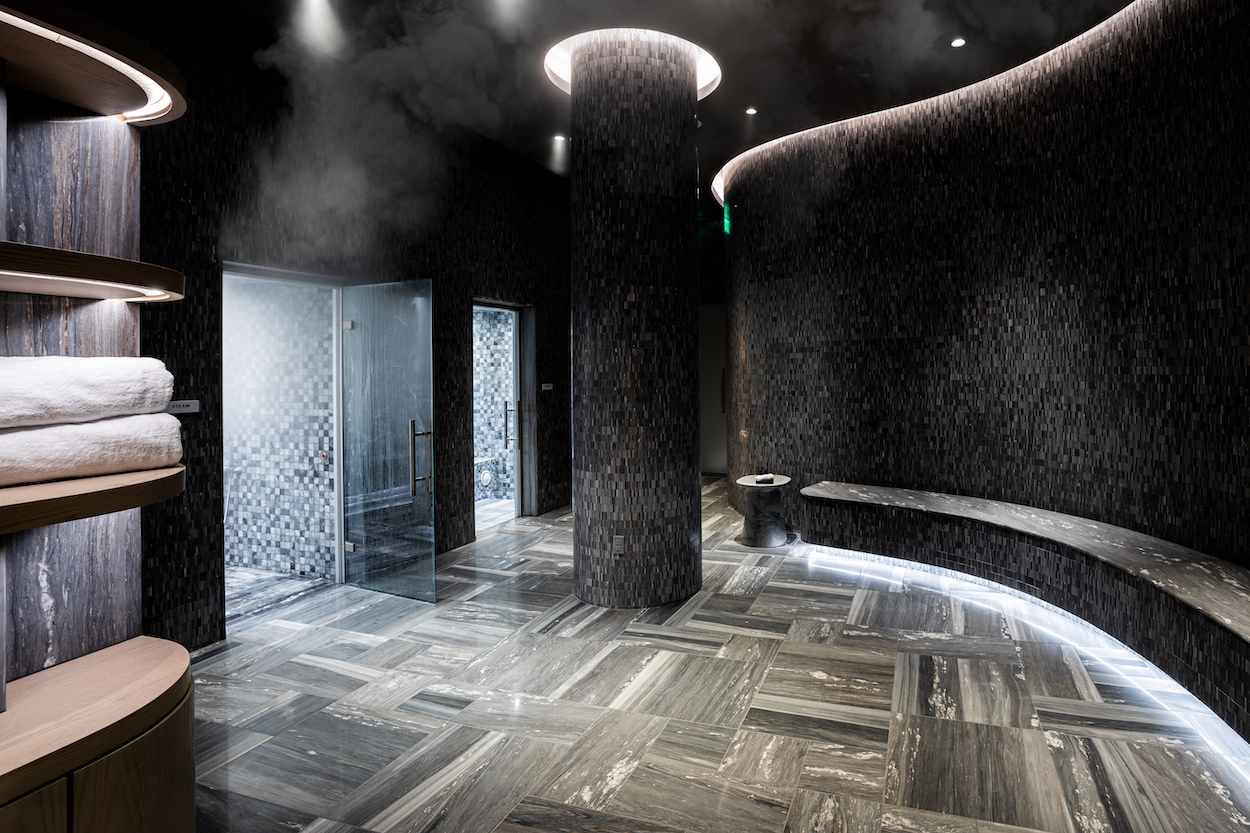This interior view of the Fairmont Century Plaza's 14,000-square-foot spa captures the luxurious seating area. At the heart of the room stands a prominent vertical column with soft, indirect lighting that highlights the ceiling. The space features beautifully tiled rooms with glass doors in the distance, which are part of the spa's amenities. On the far-left wall, four open shelves neatly display towels, adding to the room's inviting atmosphere. The walls are adorned with a mix of black and brown wood, accompanied by understated white accents and recessed lighting that casts a warm glow. The floor, an elegant mix of tan, gray, and brown parquet tiles, complements the overall upscale aesthetic. A dark brown, curved wall features an integrated seating area with subtle lighting beneath the bench, designed for ultimate comfort and relaxation. This sophisticated and well-lit image encapsulates the grandeur and tranquility of the Fairmont Century Plaza's spa seating area.